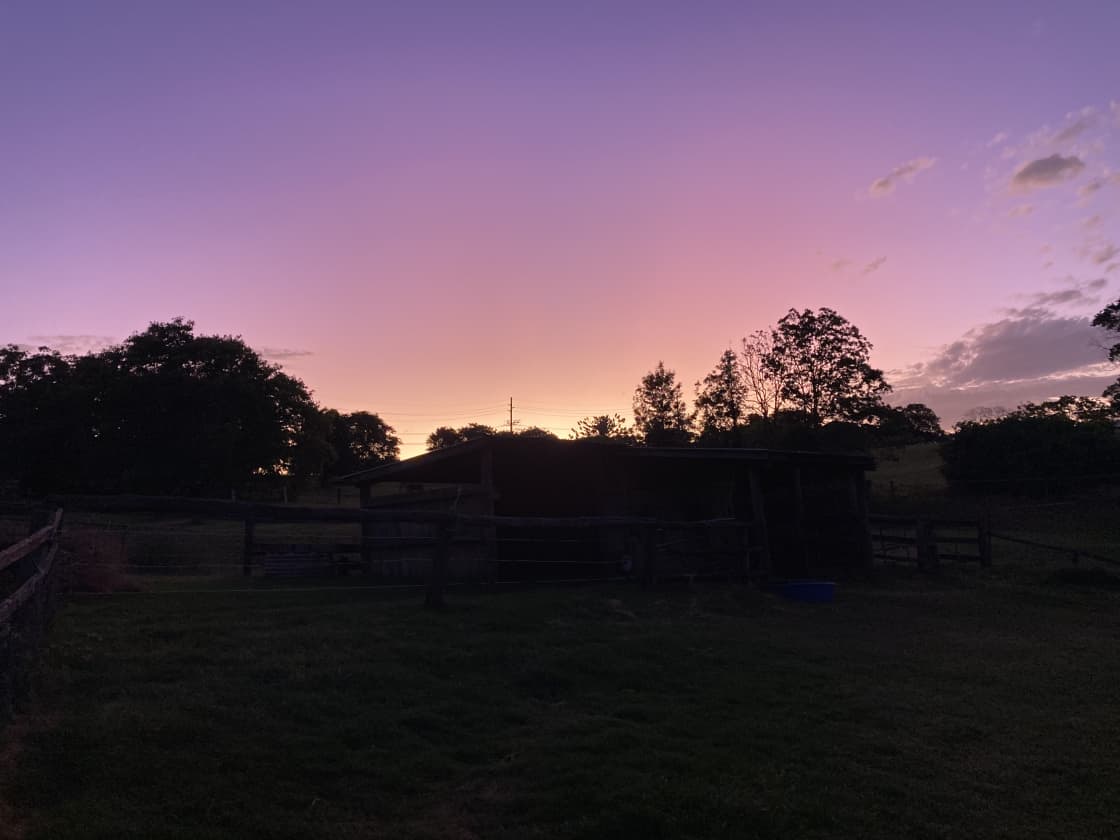The large square nighttime photograph captures a serene and vividly colored sunset. The bottom portion of the image is predominantly dark, almost black, suggesting an expanse of flat land that could either be grass or dirt. Cutting horizontally through this dark landscape is a brown wooden fence, which descends slightly on the left side. Above the fence, black silhouettes of variously shaped and sized trees populate the middle and left sections of the frame. While the trees on the left are dense, those in the middle are sparser and taller, allowing glimpses of power lines threading between them.

Dominating the top half of the photograph is a stunning, multicolored sky. It transitions gracefully from deep purple at the highest point to pink in the center, and finally to a warm yellow near the horizon where the sun has set. The vibrant sky also features feathery gray clouds on the right side, adding texture to the scene. Though the house mentioned in one caption is not visually prominent, the overall image beautifully juxtaposes the almost black silhouettes of the foreground against the radiant sunset hues of orange, pink, and blue. This striking contrast enriches the visual depth, making the photograph a captivating portrayal of a tranquil sunset landscape.